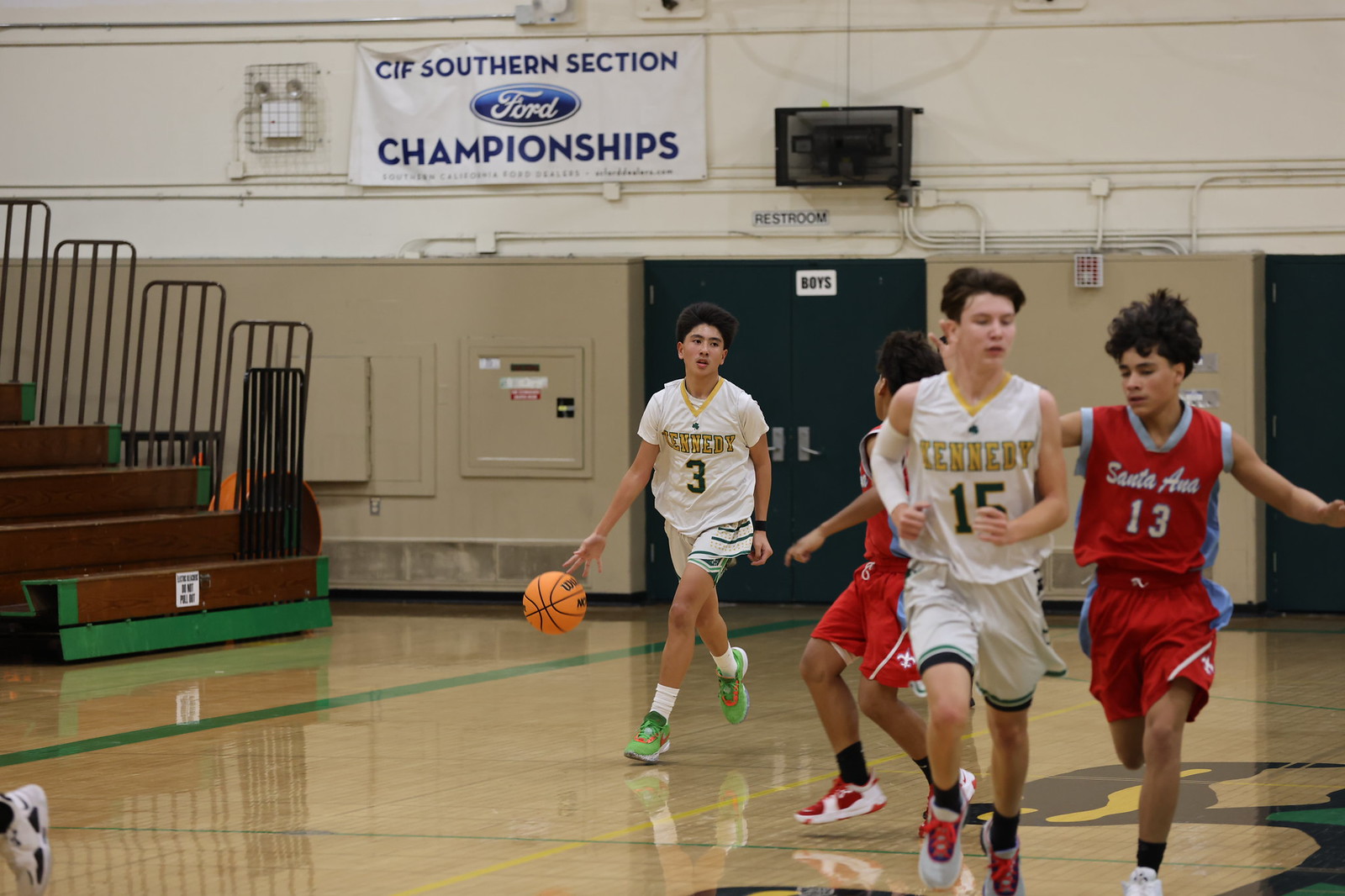This indoor photograph captures an energetic moment during a high school basketball game at the CFI Southern Section Championships, sponsored by Ford. The scene is set in a gymnasium with brown and green bleachers on the left-hand side, complete with railings, and green doors marked "boys restroom" in the background. The tan gym floor is marked with green and yellow lines.

Central to the image are four young players, all in motion, capturing an action shot. The focal player, appearing to be Asian, is dribbling an orange basketball with his right hand. He wears a white uniform with the number three and distinct green tennis shoes. Positioned to the right of the dribbler are two players in red uniforms and another in the same white uniform. Visible numbers on the players include 3, 13, and 15. The uniforms of one team are primarily white and yellow with black lettering, while the other team's are red and blue. The text "CFI Southern Section Championships" can be seen in blue and white towards the center of the background. This dynamic image captures the intensity and spirit of the game, with all players facing the photographer, though none are looking directly at the camera.